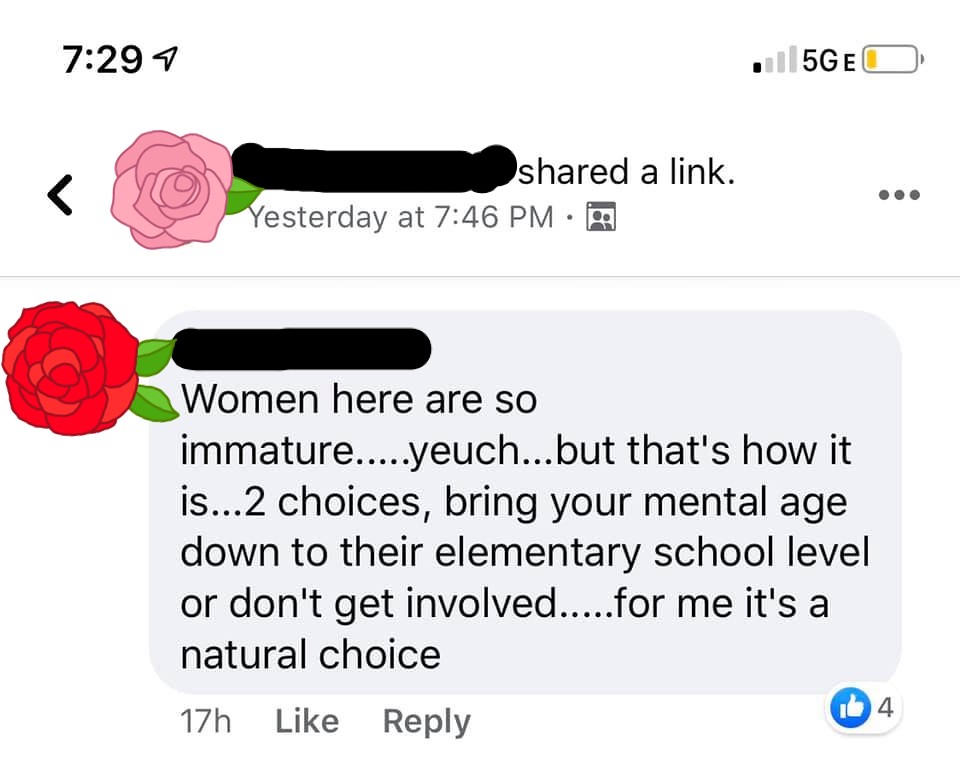This image is a color photograph, depicting a cell phone screenshot of a social media chat in square format. At the top, the phone's status bar shows the time (7:29), a diagonal right arrow, a single bar signal with a "5G" label, and a digital battery icon with one yellow bar. The first post in the chat features a user's redacted name replaced with a pink rose, indicating they shared a link yesterday at 7:46 p.m. The response thread follows, marked by a gray text box with rounded edges. The respondent's name, also redacted, appears next to a red rose symbol. Their comment reads: "Women here are so immature, yuck. But that's how it is. Two choices: bring your mental age down to their elementary school level, or don't get involved... For me, it's a natural choice." Below this comment are options to like or reply, with a blue thumbs-up icon indicating four likes.